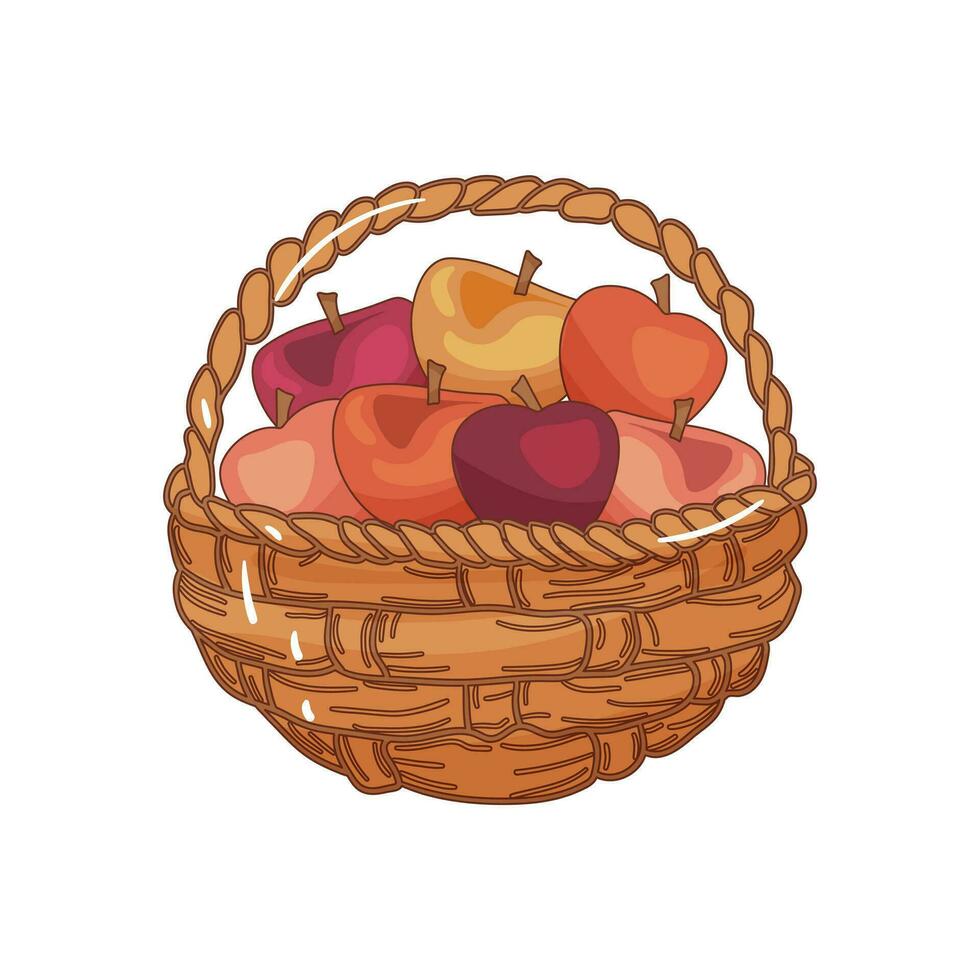This is a color illustration of a hand-drawn brown wicker basket, accentuated with white highlights to suggest texture and lighting. The basket contains around seven apples, depicted in a range of colors to capture different light reflections. The apples vary from deep red and lighter red to orange, yellow, golden, and pink-maroon hues. They are arranged in a somewhat stacked manner, with two rows: the bottom row has four apples, and the top row has three. The illustration, which appears to be digital art, is set against a stark white background, emphasizing the vibrant and diverse colors of the apples within the simplistic, woven basket.